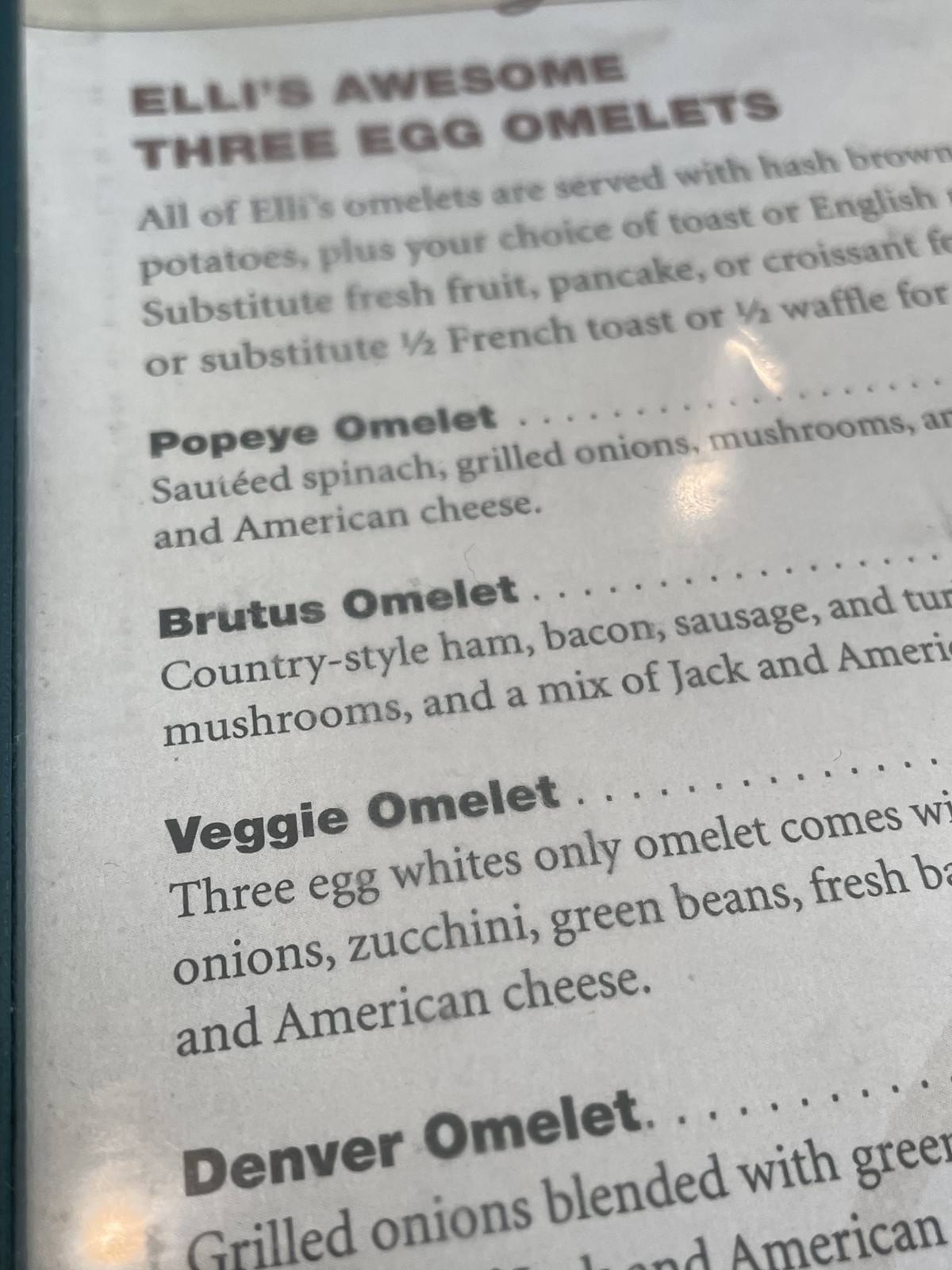This detailed black and white close-up photo of a laminated restaurant menu features a selection of "Ellie's Awesome 3 Egg Omelets." The menu, slightly blurred towards the top and with reflections visible in the lower left and upper right corners, showcases a range of richly described omelets. From bottom to top, it lists:

- **Denver Omelet** (details are partially obscured)
- **Veggie Omelet**, made with three egg whites only, including onions, zucchini, and other vegetables
- **Brutus Omelet**, featuring country-style ham, bacon, sausage, mushrooms, and a blend of Jack and American cheeses
- **Popeye Omelet**, containing sautéed spinach, grilled onions, mushrooms, and American cheese

Above these, a paragraph notes that all of Ellie's omelets are served with hash brown potatoes, with an option of toast or English muffin. Diners can substitute fresh fruit, pancake, or croissant, or opt for a half order of French toast or half a waffle instead. The detailed descriptions of each three-egg omelet emphasize their hearty and varied ingredients, underlining the unique offerings of Ellie's menu.